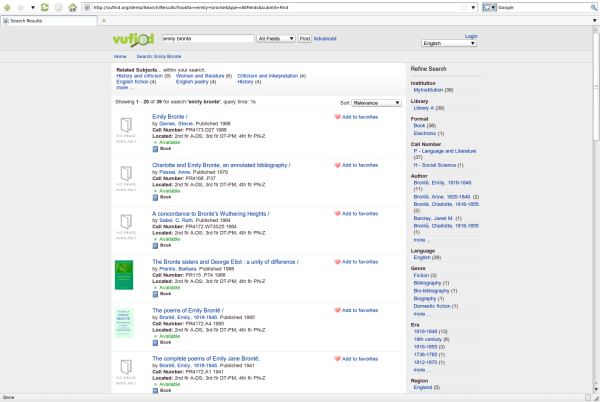This image is a detailed screenshot of a web page opened to "Vufied." The text is rather small, making it somewhat challenging to read. At the top of the page, the URL is visible. The interface is mostly gray, with a central white section where search results are displayed. 

On the upper left, there is a prominent tab labeled "Search Results." The website's logo is displayed across the top in green text, spelling out "VUFIED," with a magnifying glass over the "E." Adjacent to the logo is a search bar containing some text, likely including the term "books," accompanied by a dropdown menu set to "All Fields." Next to the dropdown are buttons labeled "Find" and "Advanced." 

On the right side of the header, there is a "Login" button and another dropdown menu set to "English." 

The search results presented in the main pane consist of a list of books. Six titles are visible, including:
1. "Emily Bronte"
2. "Charlotte and Emily Bronte: An Annotated Biography"
3. "A [Title] to Bronte’s Wuthering Heights"
4. "The Bronte Sisters"
5. "George Eliot: The Unity of Difference"
6. "The Poems of Emily Bronte"
7. "The Complete Poems of Emily Jane Bronte"

The layout clearly differentiates the search results area from the rest of the page, enhancing readability and user navigation.